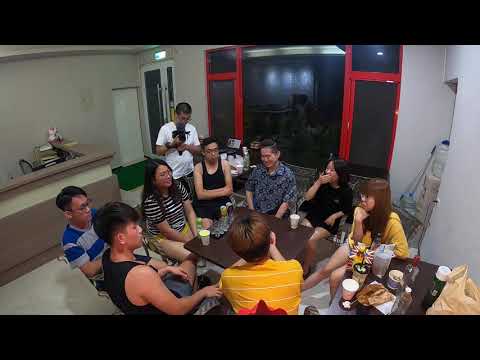In a beige-walled room that appears to be a break room, nine young adults of varying Asian descents are gathered around a small, plain brown table cluttered with cups, food, and bags. They are casually dressed and engaged in a large discussion, suggesting a meeting or event. One person stands, possibly filming with a device in hand, while the others are seated and conversing. Behind them, large windows framed in red, flanked by doors, allow natural light into the room. A shelf or desk stocked with books and some office equipment is visible in the background, hinting they might be in or near an office area.